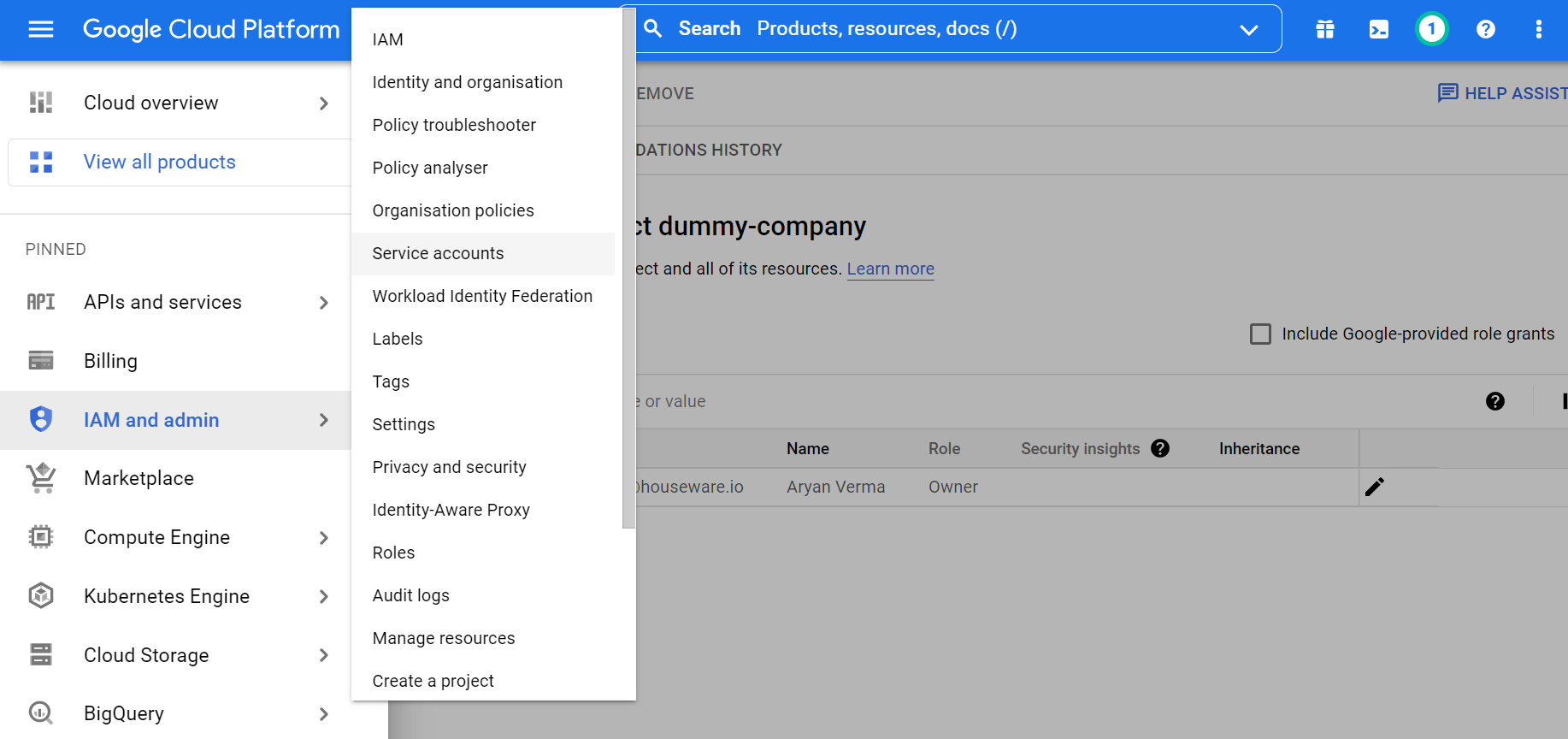This photograph captures a computer monitor displaying the Google Cloud Platform interface, most likely on a desktop or laptop screen. The top of the rectangular screen features a distinctive blue bar with white lettering that reads "Google Cloud Platform." Just below this bar, a navigation menu lists various options such as Cloud Overview, Bureau Products, and others. Some categories, like APIs and Services and Billing, are pinned for quick access. Additionally, the sidebar includes entries like IAM and Admin, Marketplace, Compute Engine, Kubernetes Engine, Cloud Storage, and BigQuery.

To the right of the sidebar, a pop-up window is open, presenting a comprehensive list of identity and organization management tools. This list includes options such as IAM, Identity and Organization, Policy Troubleshooter, Policy Analyzer, Organization Policies, Service Accounts, Workload Identity Federation, Labels, Tags, Settings, Privacy and Security, Identity-Aware Proxy, Roles, Audit Logs, Manage Resources, and Create a Playlist.

The background of the main window is slightly grayed out but still visible behind the pop-up. Notably, dark black letters spelling out "Dummy Company" are partially obscured by the pop-up. At the top of this grayed-out section is a search bar labeled "Product Resources and Docs." On the far right of the blue bar at the top, there are five white icons: a present, an unidentifiable square, a green and white circle with the number 1, a help icon with a question mark, and a three-dot menu icon.